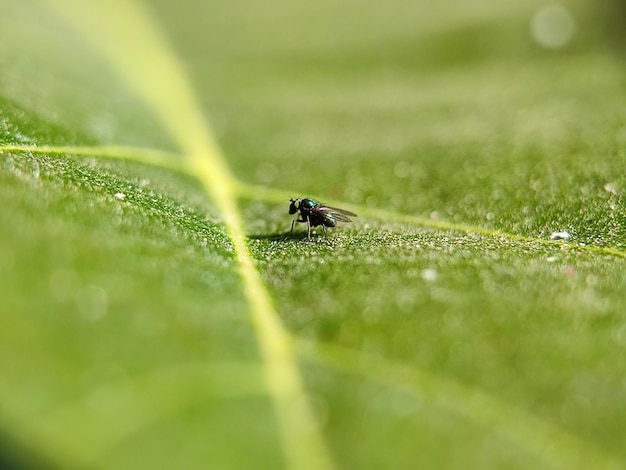This professionally taken landscape-format photograph presents a stunning macro view of a common housefly, poised on a large green leaf. Dominating the center of the image, the fly's detailed emerald-green abdomen and black wings are sharply in focus, contrasting against the subtly blurred foreground and background. Additional elements include a light green leaf emerging just left of center along the middle horizontal line, with fine surface textures akin to a cat’s tongue clearly visible due to the zoomed-in perspective. Tiny droplets of dew are scattered across the leaf, possibly indicating the fly's activity. Enhancing the composition, a faint yellowish ridge or reflection runs diagonally from the top left corner toward the center, adding depth and a tranquil ambiance to this meticulously detailed insect portrait.